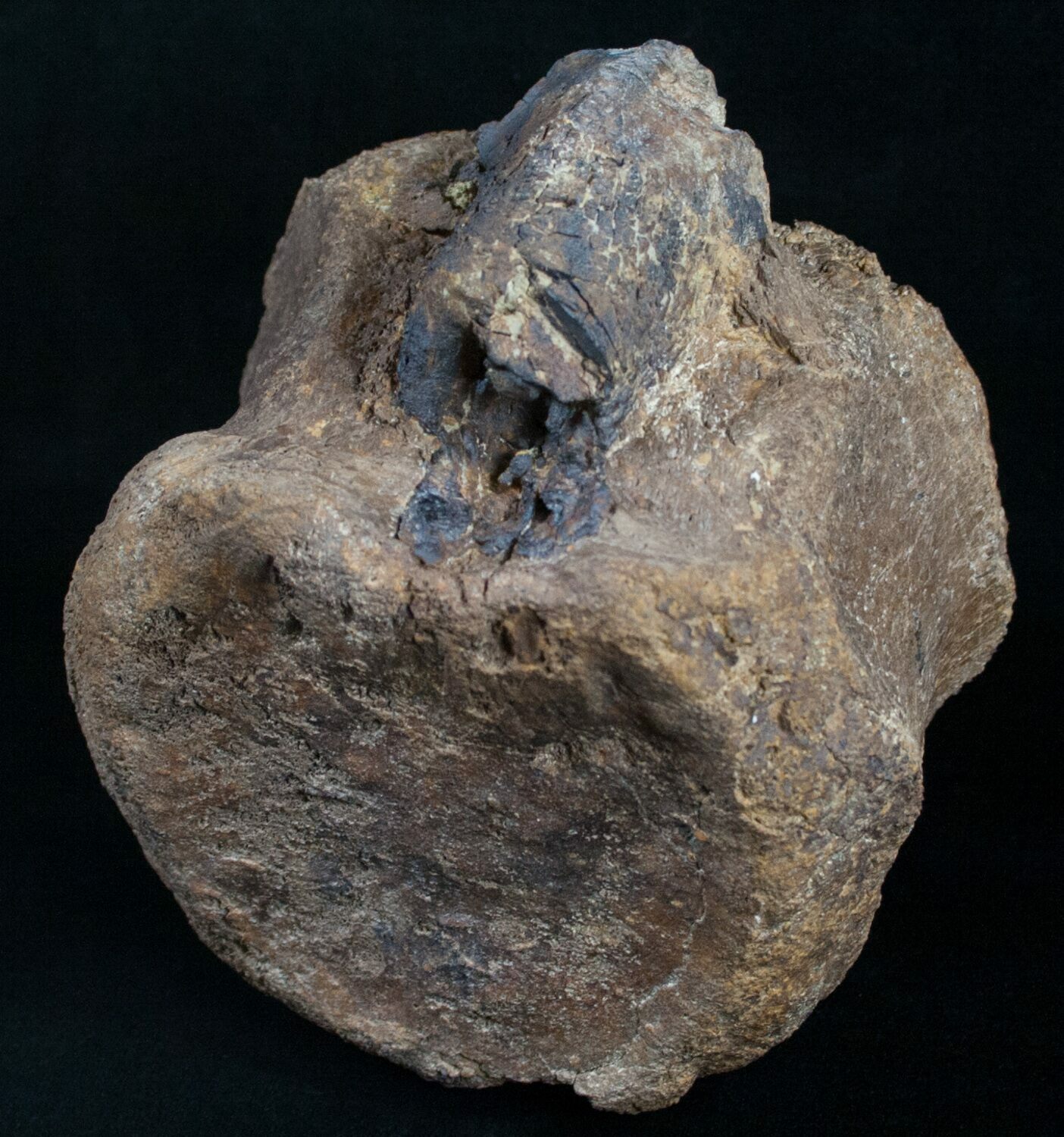The image features a large, uniquely shaped rock or potential fossil prominently positioned against a black background. The rock displays a complex texture, exhibiting a predominantly brown coloration with varying shades of black, beige, and some lighter orange sediments scattered throughout. At the top, there appears to be blackened, cracked formations, suggesting either a natural fissure or an attempt to break into the rock. The rock itself is irregularly shaped, with curved sides and an arched, almost circular bottom, and is oriented diagonally. It seems to be floating, as there is no visible surface underneath it. The overall appearance is dry, possibly aged, with a scaly texture, drawing parallels to objects of archaeological interest. This enigmatic object, while clearly textured and detailed, elicits ambiguity regarding its exact nature—potentially a fossil or a rare mineral specimen.